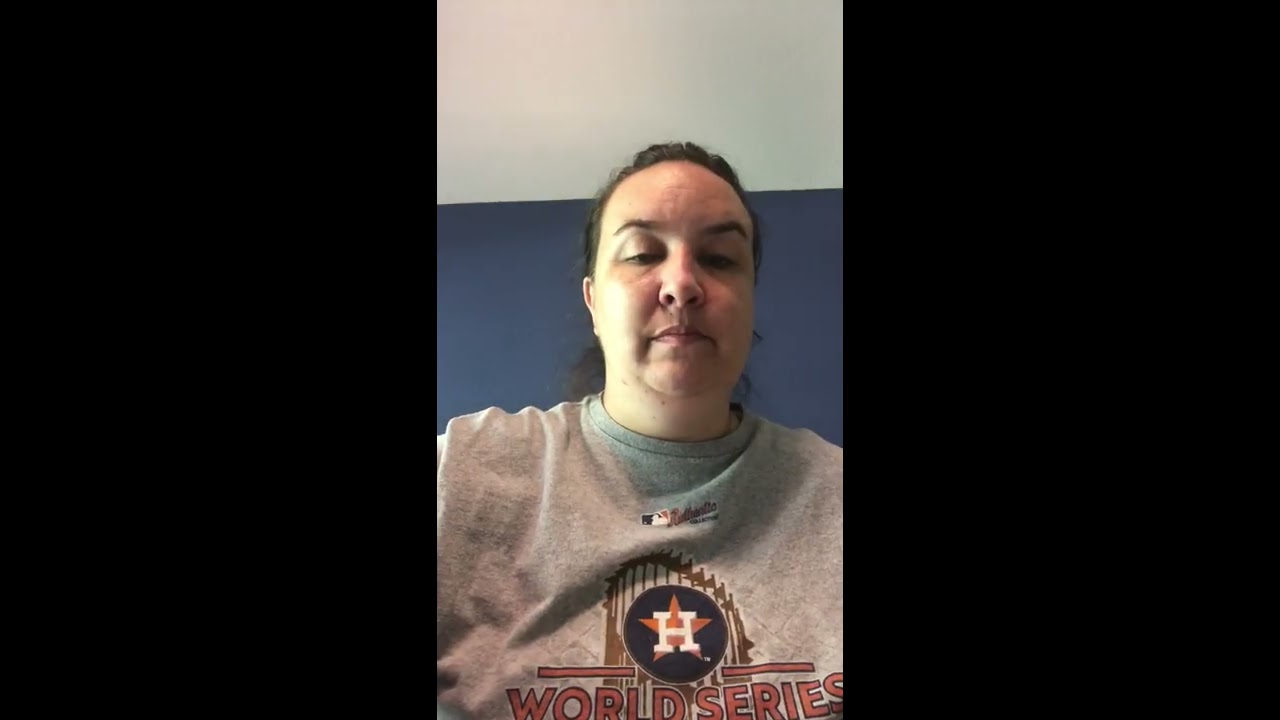In this vertically-oriented image or screenshot, the central portion features a woman of Caucasian descent, with dark brown hair pulled back into a ponytail, gazing downward as if looking at a phone. She appears to be slightly heavier set and her face is cast in shadow, with her eyes nearly closed. The woman is wearing a gray crew neck t-shirt prominently displaying "World Series" in red letters across the middle. Above the text is a distinctive circle—black or blue, depending on the lighting—with an orange or red star featuring a white 'H' in the center, representing the Houston Astros logo. There is also an MLB logo situated above this circle. The background consists of a blue wall and a white ceiling. The left and right thirds of the image are filled with black bars, giving it a bordered appearance, potentially indicating it was captured from a video or social media platform like TikTok.